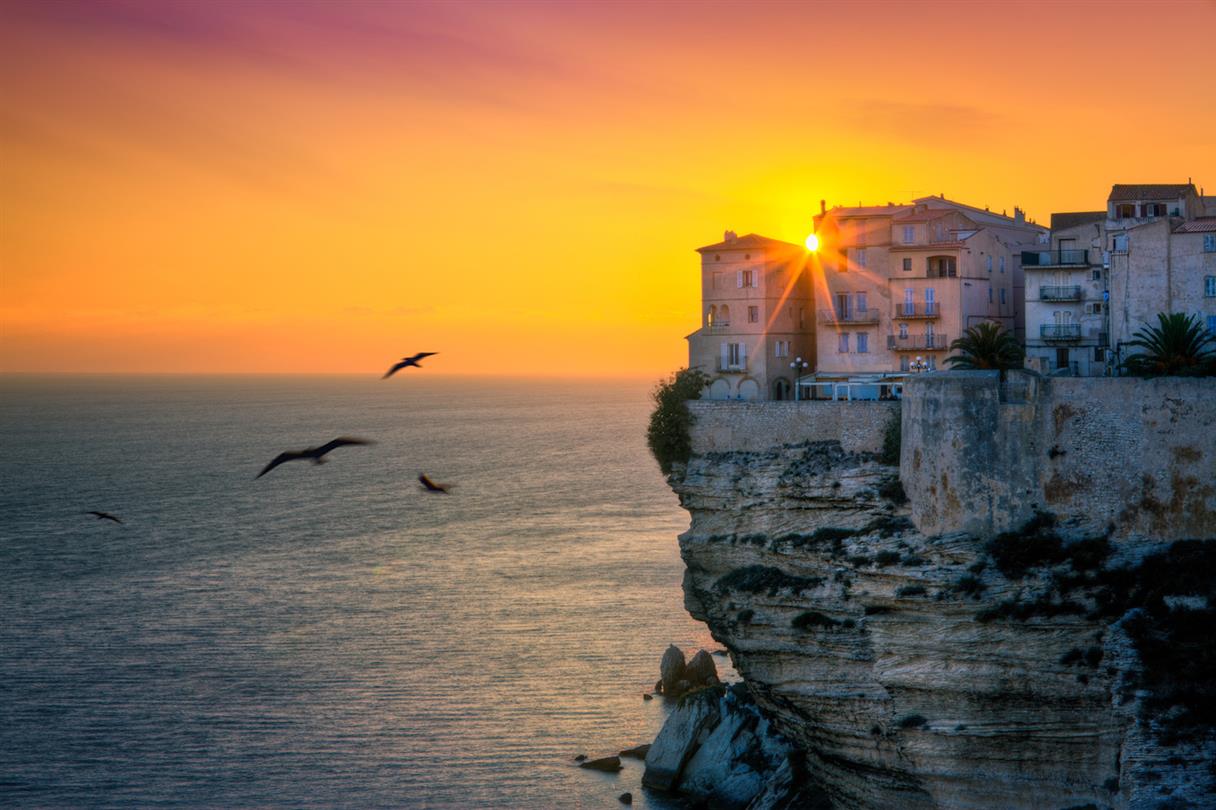The image depicts a stunning sunset over a seaside cliff. At the cliff's edge, several buildings—possibly apartments, hotels, or hostels—tower with three or four stories each, featuring multiple balconies. The structures, painted in hues of light tan, white, pink, and light brown, form a picturesque small village or townscape renowned for its idyllic ocean views. The cliff itself is rugged, revealing layers of limestone and rock formations at its base where it meets the tranquil, bluish-white ocean below. The left half of the scene showcases the vast, still sea with four silhouetted seagulls gliding over the water, backlit against a sky painted in vivid yellows, oranges, and purples. The Sun, setting behind the buildings, casts its rays between them, enhancing the serene yet dramatic atmosphere.